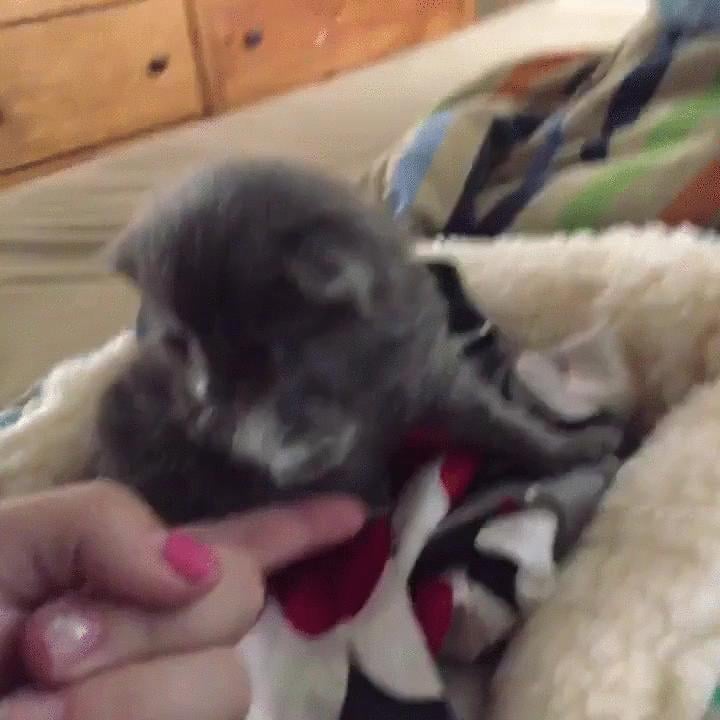In the center of this very blurry image, you can barely make out what appears to be a small kitten with predominantly dark brown fur, featuring some hints of white or gray around its chest. The kitten is situated on a fuzzy, white sherpa blanket placed on a bed covered with a cream-colored bedspread accented with green and blue stripes. In the lower left corner, a white woman's hand with pink nail polish on one finger is gently pointing at the kitten, her index finger slightly touching it. In the background, there is a closed wooden drawer, probably part of a dresser, adding some structure to the otherwise fuzzy and noisy scene. The overall image quality is very low, with significant blurriness and heavy compression, making finer details hard to distinguish.